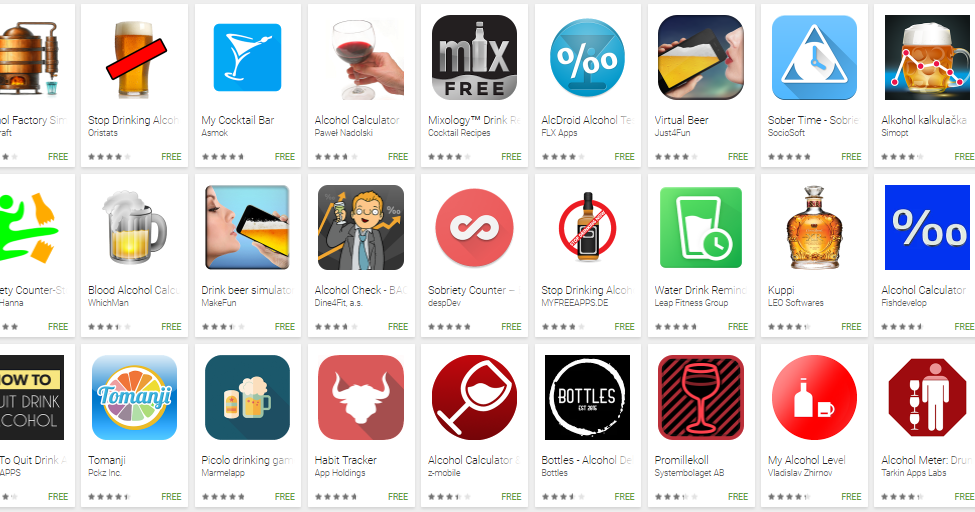Screenshot from an app store showcasing various alcohol-related applications: 

1. **Cut-off App** - The name is partially obscured.
2. **Factory Game with Alcohol Theme** - Features a barrel dispensing liquid into a cup; labeled as free.
3. **Stop Drinking Alcohol** - Displays a pint of beer with a red line through it; free.
4. **My Cocktail Bar** - Icon is blue with a white cocktail symbol; free.
5. **Alcohol Calculator** - Shows a person holding a glass of red wine; free.
6. **Mix Free - Mixology** - Available for free.
7. **AlkDroid - Alcohol Tracker** - Displays "0.00"; free.
8. **Virtual Beer** - Simulates beer drinking using phone; free.
9. **Sober Time** - Available for free.
10. **Foreign Language Alcohol App** - Title is unreadable and not in English; free.
11. **Karate Kicking Beer Bottle App** - Features a person kicking a beer bottle in half; free.
12. **Blood Alcohol Calculator** - Available for free.
13. **Drink Beer Simulator** - Available for free.
14. **Alcohol Check** - Available for free.
15. **Sobriety Counter** - Available for free.
16. **Stop Drinking Alcohol** - Available for free.
17. **Water Drink Reminder** - Available for free.
18. **Koopy/Cubby** - Available for free.
19. **Alcohol Calculator** - Available for free.
20. **How to Quit Drinking Alcohol** - Available for free.
21. **Tamanji** - Available for free.
22. **Piccolo Drinking Game** - Available for free.
23. **Habit Tracker** - Available for free.
24. **Alcohol Calculator** - Available for free.
25. **Bottles Alcohol** - Available for free.
26. **Promocol** - Available for free.
27. **Alcohol Meter** - Available for free.

First app in the list is cut off and unreadable.